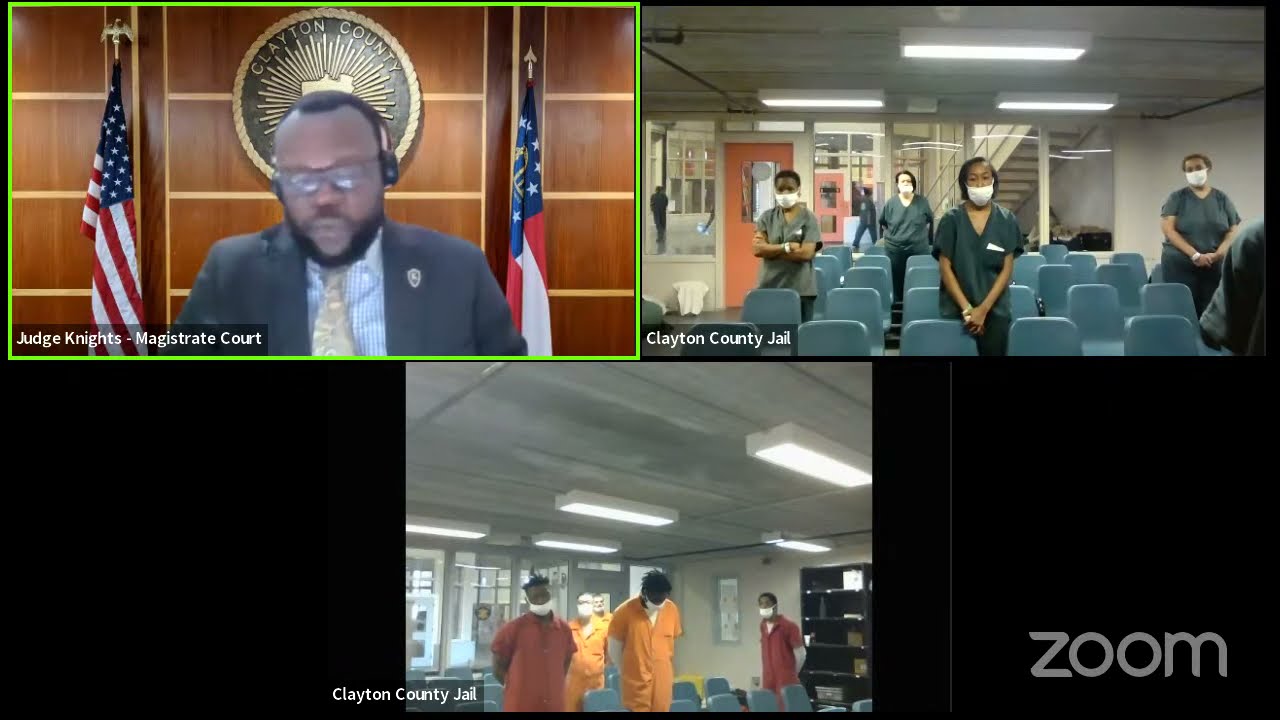The image is a composite of three video captures displayed on a black canvas, likely from a Zoom court proceeding. The top left frame is labeled "Judge Knight's Magistrate Court" and features an African-American gentleman, possibly in his early 40s, slightly balding with a beard, dressed in a gray suit, blue shirt, and yellow tie. He wears glasses and is seated, reading something. Behind him is an emblem that says "Clayton County," flanked by an American flag on his right and another flag, likely a state flag, on his left. 

The next two frames are both labeled "Clayton County Jail." The top right frame shows a room with several people, seemingly inmates, dressed in green prison attire and wearing masks. There are four individuals among mostly empty chairs. The bottom frame features a similar setting, this time with inmates in orange and yellow jumpsuits, also wearing masks. Both jail images depict individuals attending the court session via Zoom from different rooms within the jail facility.